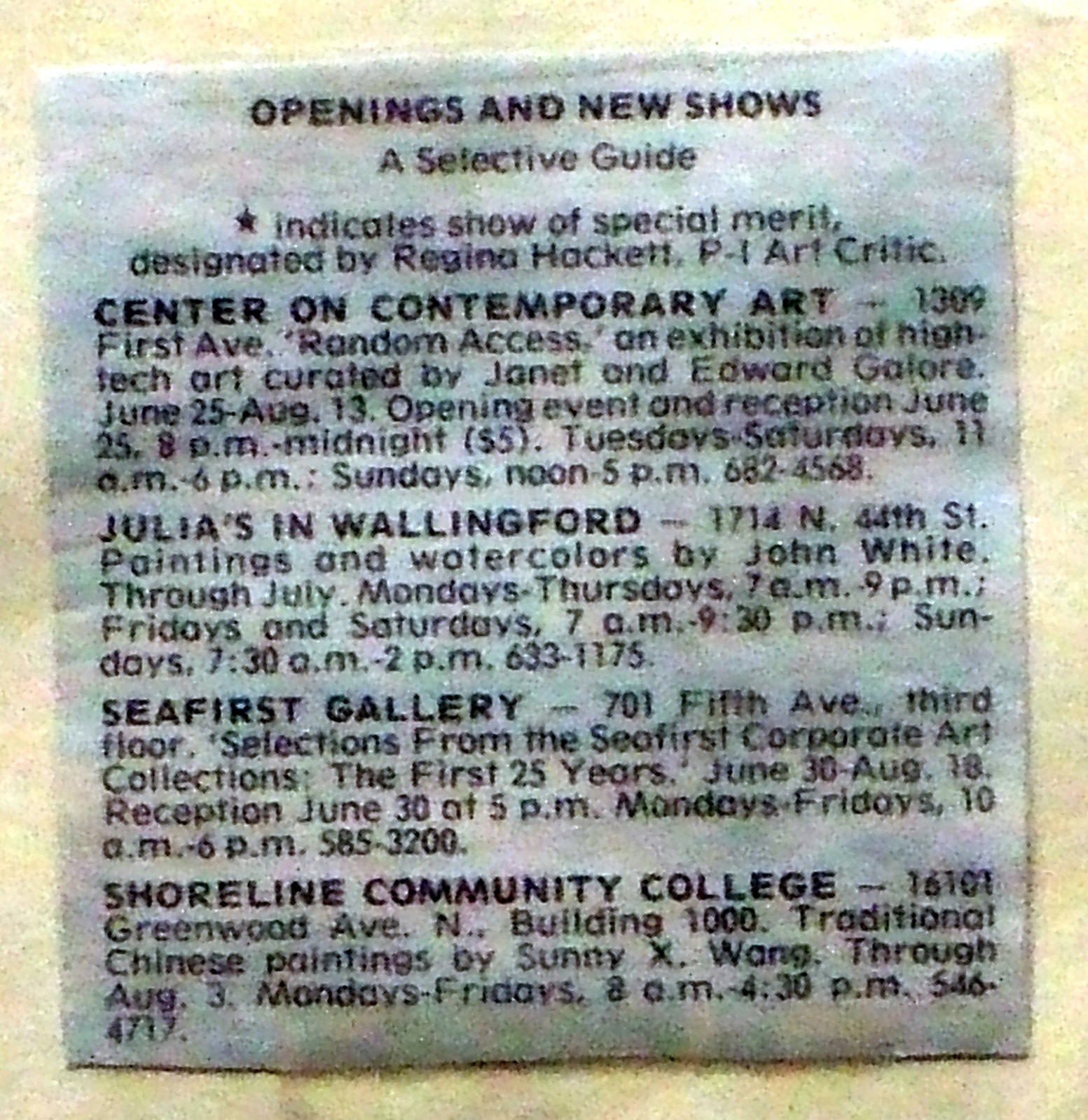The image consists of a marbleized background featuring greenish, purple, and pink hues, all blending smoothly together. Centered on this marbleized backdrop is an ivory-colored paper with a black, star symbol at the top. The bold black text on the paper reads, "Openings and New Shows, A Selective Guide," with an indication that shows of special merit are selected by Regina Hackett, P.I. Art Critic. Below this heading, there are several event listings:

1. **Center on Contemporary Art, 1309 First Avenue**:
   - **Event**: "Random Access, an exhibition of high-tech art created by Janet and Edward Galore."
   - **Dates**: June 25th to August 13th
   - **Reception**: June 25th, 8 p.m. to midnight, $5
   - **Hours**: Tuesdays to Saturdays, 11 a.m. to 6 p.m.; Sundays, Noon to 5 p.m.
   - **Contact**: 682-4568

2. **Julia's in Wallingford, 1714 North 44th Street**:
   - **Exhibit**: Paintings and watercolors by John White through July
   - **Hours**: Mondays to Thursdays, 7 a.m. to 9 p.m.; Fridays and Saturdays, 7 a.m. to 9:30 p.m.; Sundays, 7:30 a.m. to 2 p.m.
   - **Contact**: 633-1175

3. **Seafirst Gallery, 701 Fifth Avenue, Third Floor**:
   - **Exhibit**: Selections from Seafirst Corporate Art Collections, The First 25 Years
   - **Dates**: June 30th to August 18th
   - **Reception**: June 30th at 5 p.m.
   - **Hours**: Mondays to Fridays, 10 a.m. to 6 p.m.
   - **Contact**: 585-3200

4. **Shoreline Community College, 16101 Greenwood Avenue North, Building 1000**:
   - **Exhibit**: Traditional Chinese paintings by Sunny X. Wang through August 3rd
   - **Hours**: Mondays to Fridays, 8 a.m. to 4:30 p.m.
   - **Contact**: 546-4717

This detailed guide provides visitors with a comprehensive list of current and upcoming art exhibitions, including various details like dates, times, locations, and contact information.